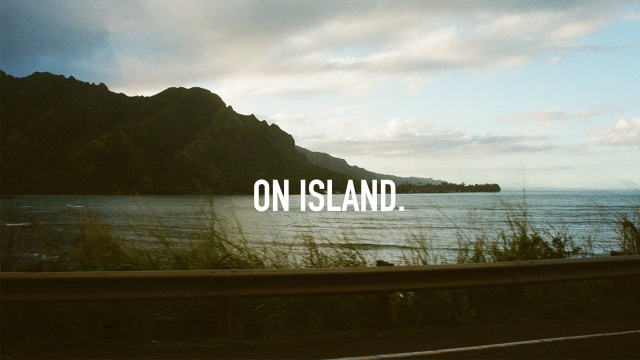The photograph titled "On Island." features a serene lakeside scene captured from the viewpoint of someone standing beside a roadside guardrail made of steel beams. In the foreground, the guardrail is visible, along with patches of grass and weeds growing along the shoreline. The setting appears to be a chilly day with the sun already set behind a distant, green, grassy hill that some might refer to as a mountain. The lake extends far into the horizon with gentle ripples spreading out across the water. The sky is mostly cloudy with hints of residual sunlight evident behind the clouds, adding a calm and somewhat somber atmosphere to the scene. The phrase "ON ISLAND." is prominently displayed in bold, traditional white font across the middle of the image, slightly towards the bottom, drawing focus to the hill and water beyond.